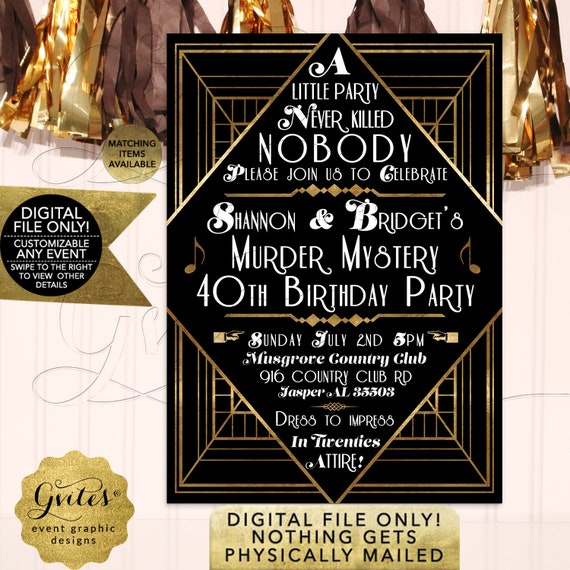This image is a digital invitation poster featuring a stylish, vintage theme inspired by the Roaring Twenties. Central to the poster is a sleek black rectangle bordered by golden lines, containing elegant white text that reads: "A little party never killed nobody. Please join us to celebrate Shannon and Bridget's murder mystery 40th birthday party." The event details specify that it will be held on Sunday, July 2nd, at 5 p.m. at the Miss Grower Country Club, located at 916 Country Club Road, Jasper, AL 35503. Attendees are encouraged to dress to impress in 1920s attire. Below the central rectangle, additional text in black emphasizes that this is a digital file only and that nothing will be physically mailed. Surrounding the central rectangle, the poster's background features a design with shiny ribbons in brown and golden colors, enhancing the vintage ambiance of the invitation.